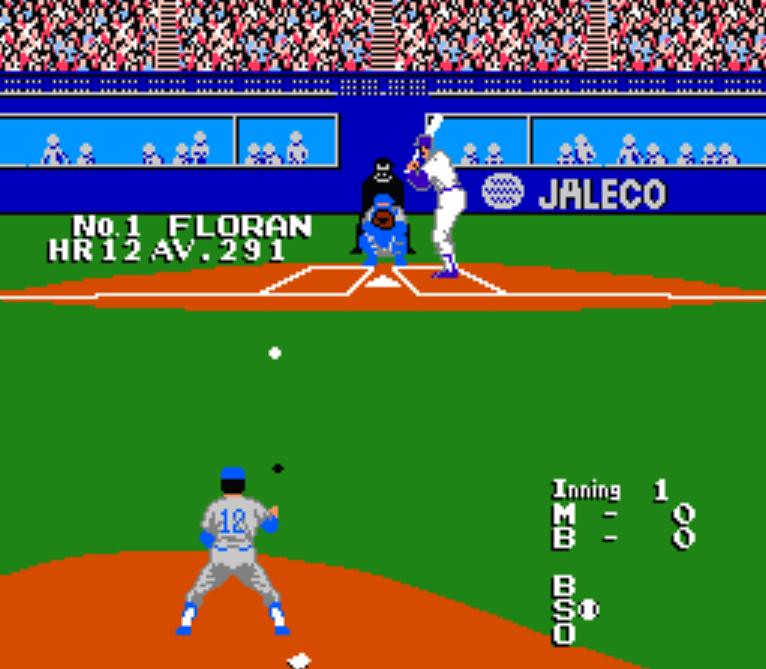The image depicts a vintage 1980s baseball video game, likely from the late 80s. The game screen prominently displays the logo "Jaleco" in the background, possibly positioned near the dugout areas. The graphics are pixelated, reflecting the era but remain clear enough to discern the game's elements. The stadium is packed with a diverse crowd dressed predominantly in red, blue, and white. The scene features three rows of stairs, indicating a multi-tiered seating arrangement. 

On the field, the pitcher, clad in blue and silver, is in the midst of throwing a pitch, while the opposing team, dressed in white and blue, is ready for the play. Notably, the batter and catcher are in their respective positions, with an umpire overseeing the action. The player "Florin" is indicated as number one. At the top of the screen, the game shows it is the first inning with no runs scored yet.